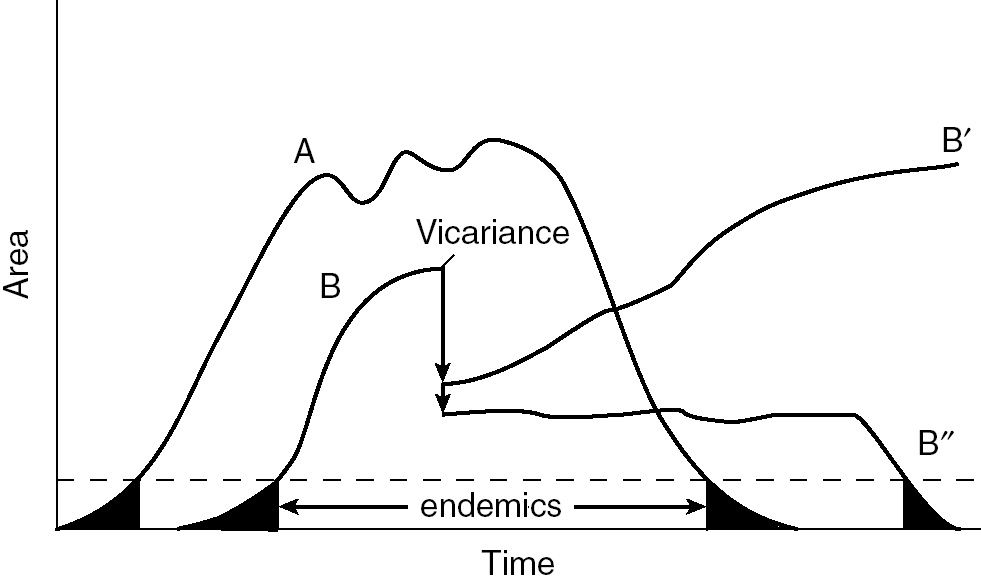The image is a detailed graph with a white background, presenting a complex relationship between area and time. The vertical axis on the left is labeled "Area," and the horizontal axis at the base is labeled "Time." Near the bottom, slightly above the base, there is a dotted line stretching across the graph, below which the word "Endemics" is printed. The graph features two main lines: Line A and Line B. Line A starts at zero and rises to over halfway up the graph surface before returning to zero, forming a bell-shaped curve. Line B also begins at zero, but it rapidly rises and then sharply falls. Within the Line B area, there are two alternative trajectories: B' (B prime), which rises, and B'' (B double prime), which returns downward in a bell-shaped manner. Arrows and labels in black text point to various features within the graph, with the word "Vicariance" centered near the middle of the graph to indicate a specific section associated with Line B. Despite the detailed layout, the graph lacks numerical values and contextual information, making it challenging to fully interpret the data presented. The rest of the background remains plain and uncluttered.